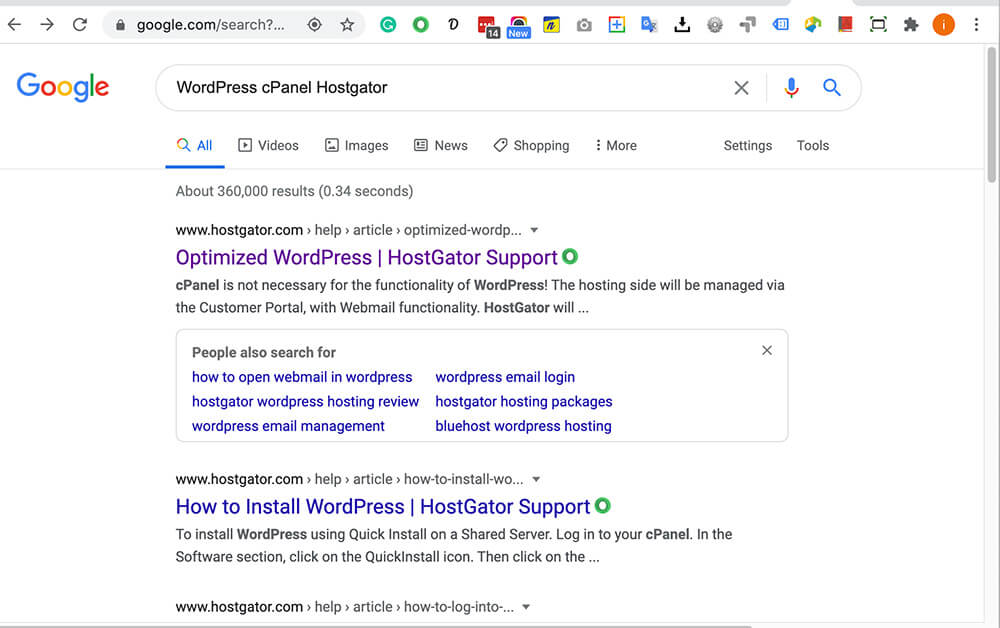A detailed description of a Google search results page is captured in this image. The screenshot includes the search bar at the top, featuring the URL "google.com/search?" with a padlock icon, navigation arrows, a refresh button, and a series of symbols. The symbols include a green button with a white 'G' representing Google, a green circle, an unidentifiable pear-shaped icon, a red box with white text, a black box with white '14', and an orange segment beside a black circle with an adjacent blue text box labeled 'new'. 

At the upper left corner, the colorful Google logo prominently displays its blue 'G', a red 'o', a yellow 'o', a blue 'g', a green 'l', and a red 'e'. The search box below contains the search terms "WordPress, cPanel, HostGator," alongside the search control icons: an 'X', a microphone, and a magnifying glass.

The search results reveal approximately 360,000 results in 0.34 seconds, with the first result coming from www.hostgator.com, titled "Optimize WordPress HostGator Support." The link appears in purple, indicating it has been previously clicked. Below, six related search suggestions are visible under "People also searched for."

The second result, "How to Install WordPress HostGator Support" from hostgator.com, appears in blue, indicating it has not yet been clicked. The third visible result begins with "www.hostgator.com, help, article, how to log into...," but the rest of the text is truncated.

On the far right of the image, a gray progress bar is visible, suggesting the ability to scroll through the search results, though the bar is currently locked at the top of the viewable area.

This comprehensive depiction of a Google search page effectively communicates the essential details of the search query and results layout.